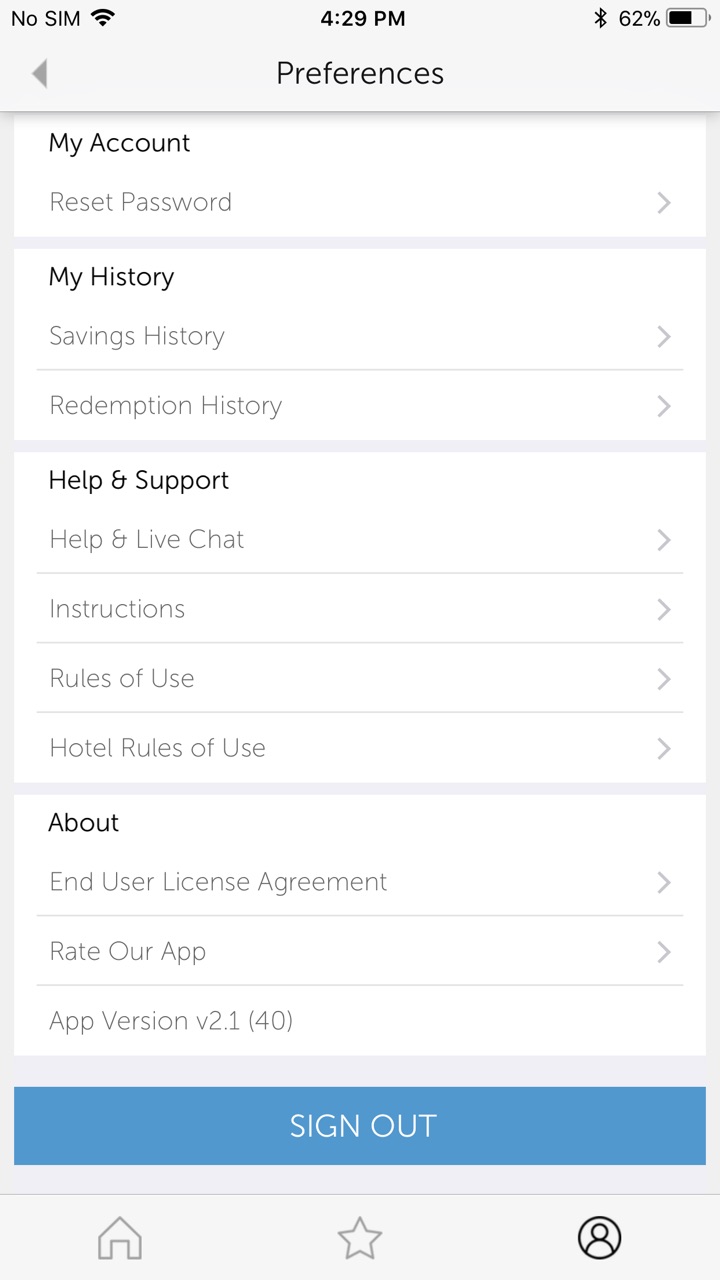Screenshot of a smartphone interface showing various settings and information:

- **Top section**: 
  - Notification reading "No SIM" in bold black lettering on a gray background.
  - Internet access icon.
  - Time displayed as 4:29 PM at the center.
  - Battery life indicator at 62% on the far right.

- **Mid-section**:
  - A banner with a back button on the left.
  - The word "Preferences" in gray at the center.

- **Main body**: 
  - Multiple white background boxes stacked vertically, each containing specific settings or information.
  - **First Box**: 
    - "My Account" in dark gray text.
  - **Second Box**: 
    - "Reset Password" in dark gray with a right-facing arrow.
  - **Third Box**: 
    - "My History" in dark gray.
    - Sub-items listed underneath in lighter gray:
      - Savings History
      - Redemption History
  - **Fourth Box**:
    - "Help and Support" in dark gray.
    - Sub-items listed underneath in lighter gray:
      - Help
      - Live Chat
      - Instructions
      - Terms of Use
  - **Fifth Box**:
    - "About" in dark gray.
    - Sub-items listed underneath in lighter gray:
      - End User License Agreement
      - App Version 21 (40)
    - A blue "Sign Out" button at the bottom.

This detailed and structured caption provides a comprehensive description of the interface shown in the screenshot.